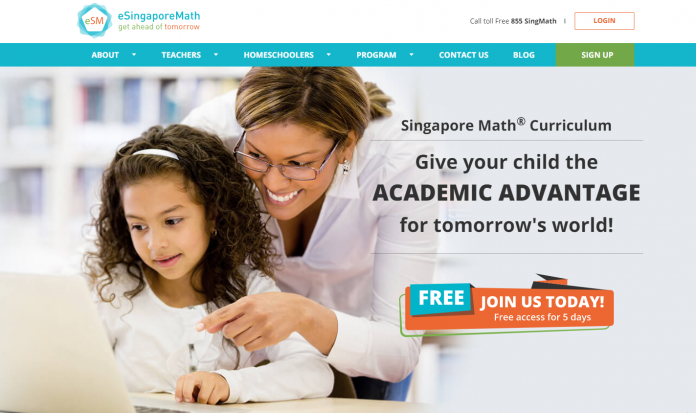**Website Home Page Description**

At the top of the home page, there's a white header occupying about an inch of vertical space. Below this white header, approximately an inch from the left, there is a line that stretches horizontally across the bottom. This line has varied patterns, which include slight upward-right and upward-left movements, peaking towards the center.

The background is primarily white with a subtle blue border enclosing a logo. The logo features a small green 'E', followed by a large red 'S' and 'M'. Outside the logo, to its right, there is a small blue 'E' accompanied by the text "Singapore Math" in black. Below this text, there is a tagline that reads "Get Ahead of Tomorrow", with 'Tomorrow' emphasized in red.

On the right side of the header, approximately an inch inward, there's a white tab with a red border that reads "Log in". To the left of this tab, contact information, specifically a phone number, is present. Below this, a navigation bar with a blue border coming from the left side houses several dropdown menus labeled "About", "Teachers", "Homeschoolers", and "Program", along with "Contact Us" and "Blog". There's also a green tab saying "Sign Up".

Centrally located below this navigation area, there is a photograph featuring a smiling woman with brownish-blonde hair pulled back, wearing glasses and a long white sleeve shirt. She is leaning forward, seemingly engaged with a young girl beside her. The girl, with shoulder-length brown hair, is focused intently on a white laptop located in the bottom left corner of the image. The girl’s left hand is resting on the keyboard, while the woman’s arm reaches across the girl's body to point at the computer screen.

To the right of the woman’s head, in black text, it says "Singapore Math Curriculum". Below this text is a thin line, and then larger black letters read "Give your child the", with "Academic Advantage" emphasized in all bolded capital letters. Continuing in regular bolded black text, it concludes with "for tomorrow’s world".

Beneath this statement, a prominent orange banner spans the width of the bottom part of the page. At the top left corner of this banner, a blue tab labeled "Free" in white text grabs attention. The banner itself encourages visitors to "Join us today", and underneath this call to action, smaller white text offers "Free access for five days".